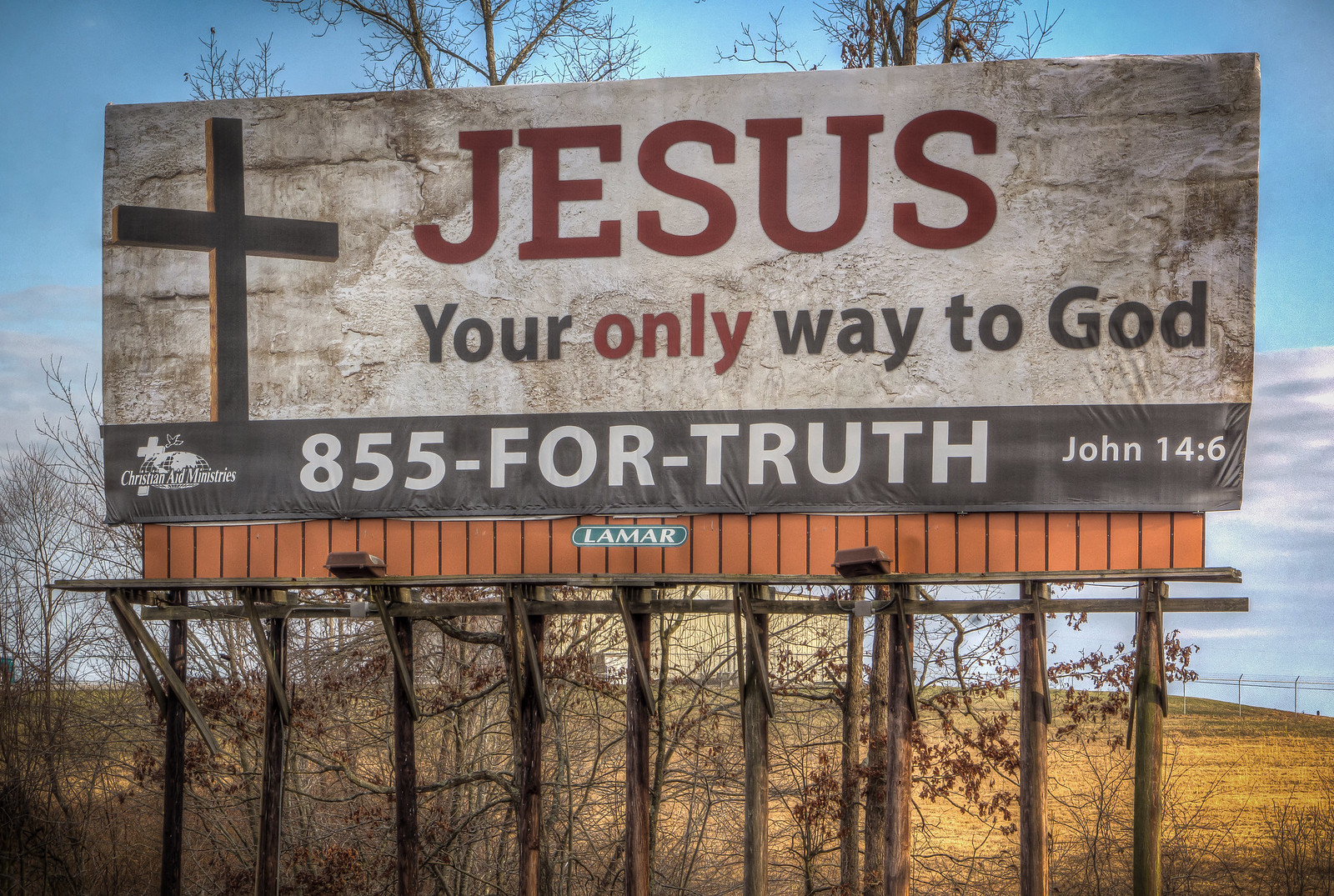The image features a prominent billboard situated along the roadside, surrounded by an expanse of barren, lifeless trees and dry, withered grass, evoking a late autumn atmosphere where the leaves have fallen, leaving an intricate network of slender branches exposed. Bathed in the bright light of a sunny day, the billboard stands as the central focus of the scene, displaying a bold message: "Jesus, your only way to God." In the lower corner of the billboard, the Christian Act Ministries logo is visible, accompanied by the text "855 FOR TRUTH, John 14:6." Below the message, another logo identifies Lamar as the billboard company. The image is a close-up shot, emphasizing the stark contrast between the vibrant message and the desolate surroundings, with no other significant elements present in the frame.